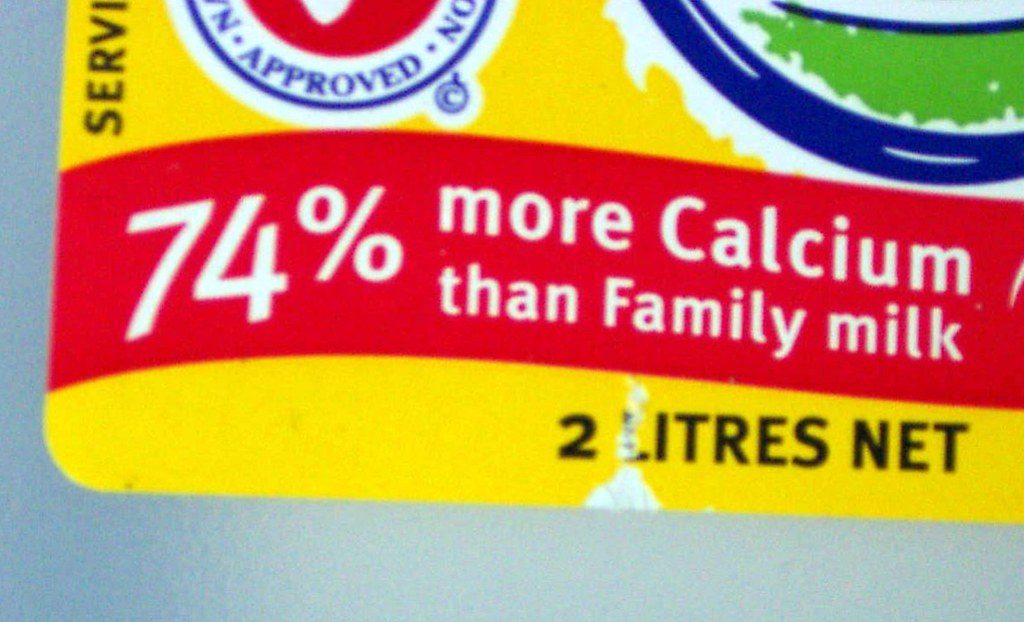This image captures a partial view of a product label, predominantly yellow in color. A distinctive red strip lines the bottom of the label, prominently stating "74% more calcium than family milk." Beneath this message, the label indicates the net weight as "2 liters." Above the red strip, part of a round circle logo is visible, along with the associated text "approved" and a small circle with a 'C', signifying copyright. Running along the sides of the label are the letters "S-E-R-V." The upper portion of the label showcases a blue design overlaying a white design, topped by a green color stripe, and another blue line higher up.